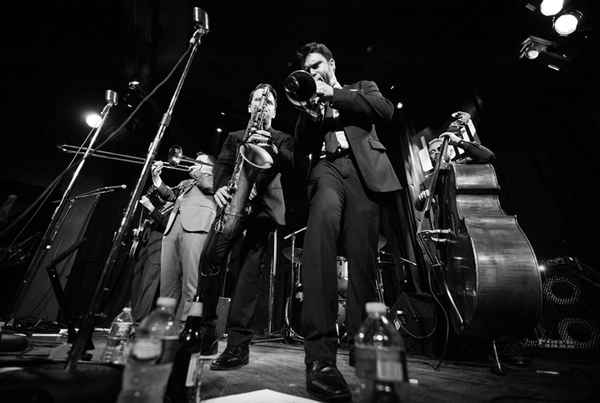In this evocative black-and-white photograph, a band is captured mid-performance, bringing a sense of energy and nostalgia. The band members, suited up in precisely tailored attire, command attention with their crisp jackets, ties, formal suit pants, and slightly shiny black leather shoes. While most of the suits are a uniform dark color, one stands out in a lighter shade of grey.

Each musician is deeply engrossed in their craft: one plays a trumpet, another wields a saxophone, a third handles a trombone, and a fourth is engaged with what appears to be an upright bass. In the background, partially obscured, a fifth musician is playing an instrument that is likely a guitar or something similar. The group stands confidently on a stage, illuminated by strategic lighting that punctuates the otherwise dark backdrop. Scattered water bottles in the foreground hint at the intensity of their performance and the practical needs of the performers.